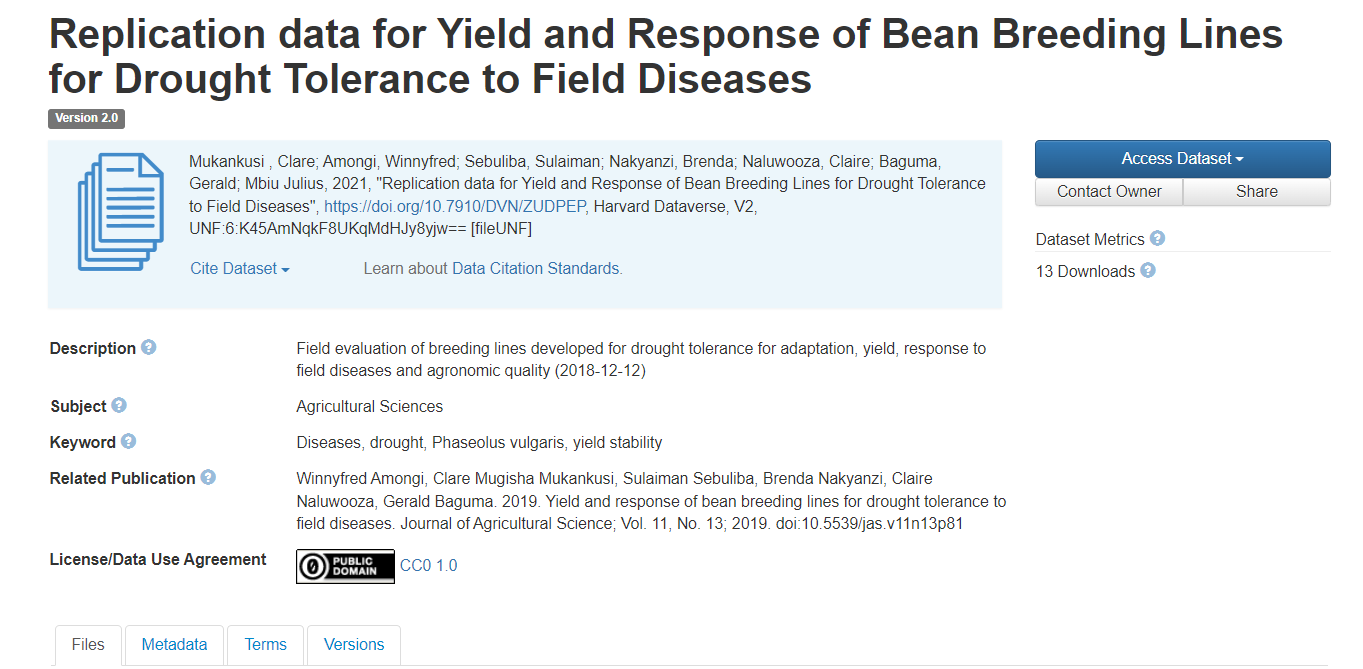The image is a detailed, horizontal rectangular graphic titled "Replication Data for Yield and Response of BEAN Breeding Lines for Drought Tolerance to Field Diseases." This title is prominently displayed at the top in bold black font. Beneath the title, there's a light blue band containing a small logo and some text in black font. The logo resembles a stack of papers, characterized by a piece of paper with a folded corner, blue horizontal lines, blue edges, and overlapping sheets. The text next to the logo is difficult to decipher.

On the left side of the light blue area, several keywords are listed in bold black font, each accompanied by a blue circle containing a white question mark. The first keyword is "Description," followed by an explanation in regular black font: "Field evaluation of breeding lines developed for drought tolerance, adaptation, yield response to field diseases, and agronomic quality." The second keyword is "Subject," with the corresponding text indicating "Architectural Sciences." The third keyword is "Keyword," with associated terms listed as "Diseases, Drought, Facetious, Vulgars, Yield Stability."

Further down, under the section marked "Related Publication," the text mentions a publication title, "Yield and Response of Bean Breeding Lines for Drought Tolerance to Field Diseases," published in the Journal of Agricultural Science. 

At the bottom of the light blue section, the terms "License / Data Use Agreement" are noted alongside a black rectangle containing the text "Public Domain" in white lettering.

The very bottom of the image features a line of options in blue font: "Files," "Metadata," "Terms," and "Versions," each within its own horizontal box separated by light grey lines. Notably, "Files" is not in blue font.

On the right side, near the top, there's a horizontal blue box with white font and a pull-down menu reading "Access Dataset." Below this are two buttons: "Contact Owner" on the left and "Share" on the right, both in black and grey boxes, separated by a thin line. Additionally, the text "Data Metrics" appears, noting "13 Downloads."